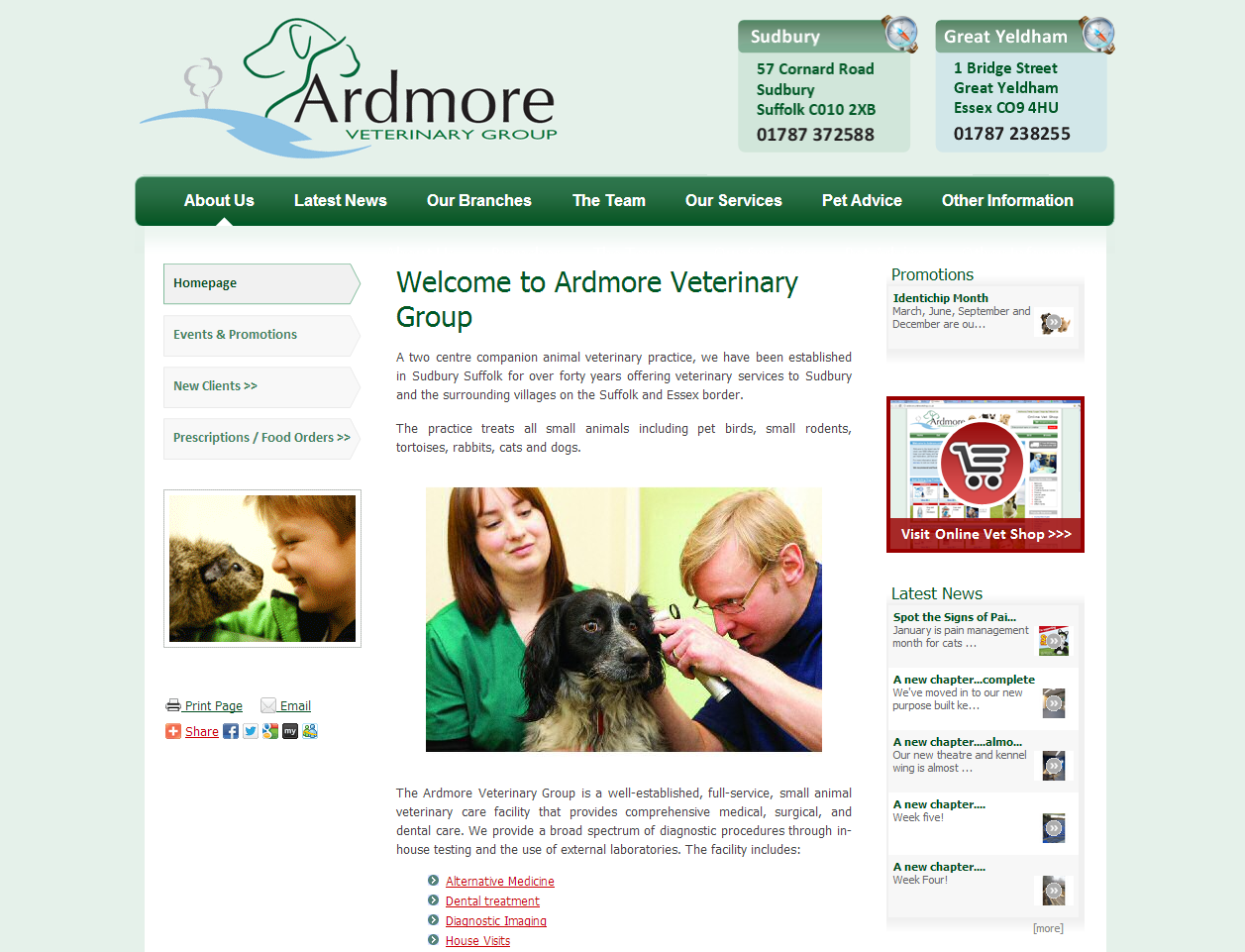**Caption:**

The webpage for Ardmore Veterinary Group, spelled A-R-D-M-O-R-E, features a comprehensive 'About Us' section. The logo combines a lion, resembling a dog, beside a tree and a path. The page borders are in a light gray and pastel green color scheme. Two highlighted boxes display information with watch icons, detailing their branches:

1. Sudbury: 59-57 Cornard Road, Sudbury, Suffolk, CO10 2XB, Phone: 01787 372588
2. Great Yeldam: 1 Bridge Street, Great Yeldam, Essex, CO9 4HU, Phone: 01787 238255

Navigational tabs include About Us, Latest News, Our Branches, The Team, Our Services, Pet Advice, and other information. To the left, there's a menu with Home, Events, Promotions, New Clients, and Subscription/Food Orders options. Below this is a photograph of a young boy smiling at a small mammal, possibly a rabbit or guinea pig.

Interactive icons for printing, emailing, and sharing are featured, along with logos for Facebook, Twitter, Google Plus, and two other indistinguishable platforms.

The main content welcomes visitors to the veterinary group, accompanied by an image of a vet examining a dog's ear while its owner holds it. Both individuals appear to be of European descent, and the dog might be a Cocker Spaniel.

Further links provide information on Alternative Medicine, Dental Treatment, Diagnostic Imaging, and House Vets, alongside promotions like IndyChip available in March, June, September, and December. A shopping cart icon leads to the online vet shop. 

The Latest News section features headlines such as "Spot Signs of PAI," "A New Chapter," and other ongoing updates, each followed by ellipses, indicating further content.